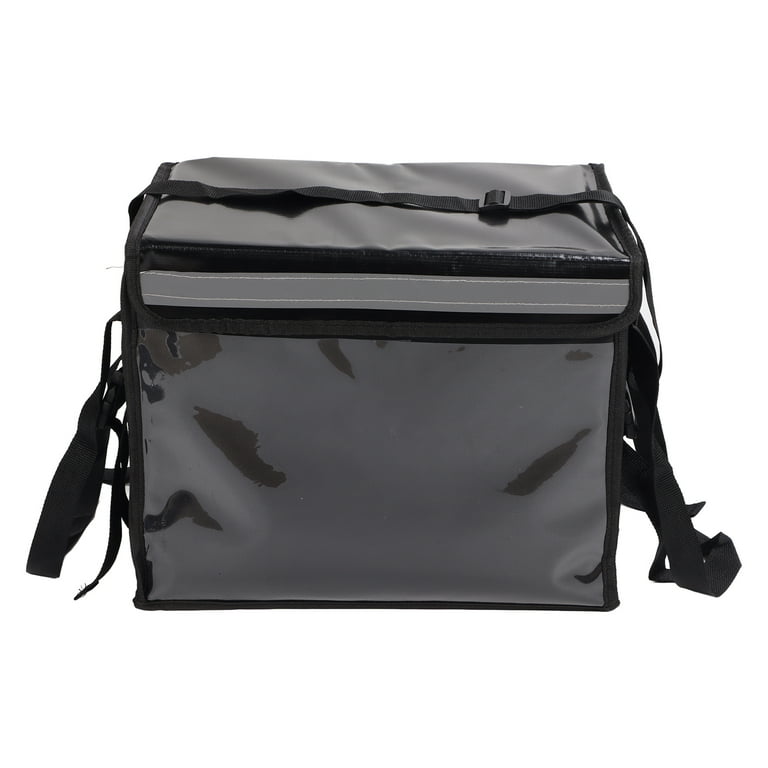The photograph shows a horizontally aligned, rectangular storage box, likely designed for keeping food cold, with distinctive black and grey paneling. The box appears to be made of backpack-like, woven plastic fibers, and is covered in a clear, glossy plastic layer. Black straps hang down from both the left and right sides, while another black strap spans the top horizontally, equipped with a square-shaped, sliding plastic adjuster. The side and front surfaces are primarily grey but maintain a shiny, plastic-coated appearance, potentially giving the impression of a transparent layer over black paneling. A noticeable feature includes a centimeter-high flap at the top, approximately 10 centimeters across, outlined in black trim. The black trimming is consistent around all edges of the box, reinforcing its durable construction. The box’s design echoes a style that could have been from 20 years ago to contemporary times.